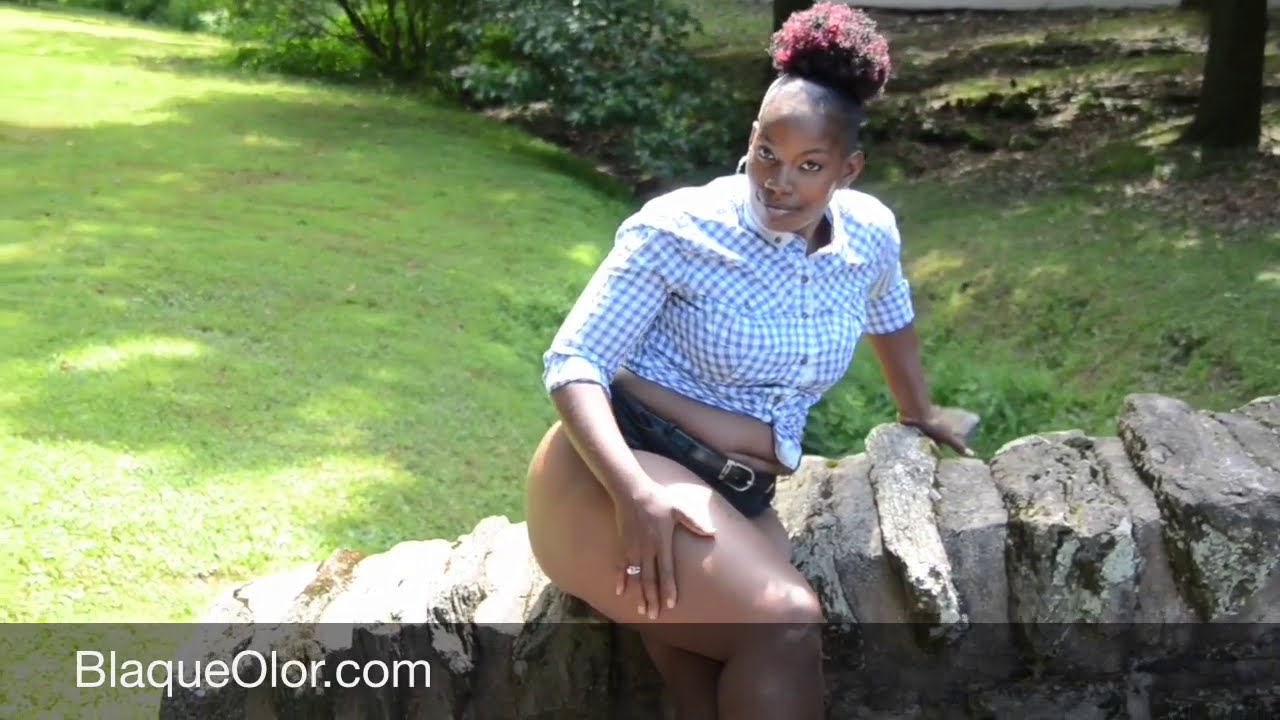In this image, a zaftig African American woman is posing outdoors against a stone wall. She is wearing a blue and white checkered picnic shirt that is tied to reveal her midriff and very small black shorts, showcasing her bare legs. The woman's hair is dyed pinkish-black and styled in a bun, while she accentuates the look with big hoop earrings and a ring on one of her fingers. Smiling radiantly at the camera, she appears to be advertising for BlackAllure.com, as indicated in the bottom left corner of the image. Midday sunlight highlights her features, suggesting it is around noon. The background consists of lush greenery, including closely cropped grass, several trees, bushes, and numerous leaves scattered on the ground, indicating a park or forest setting.